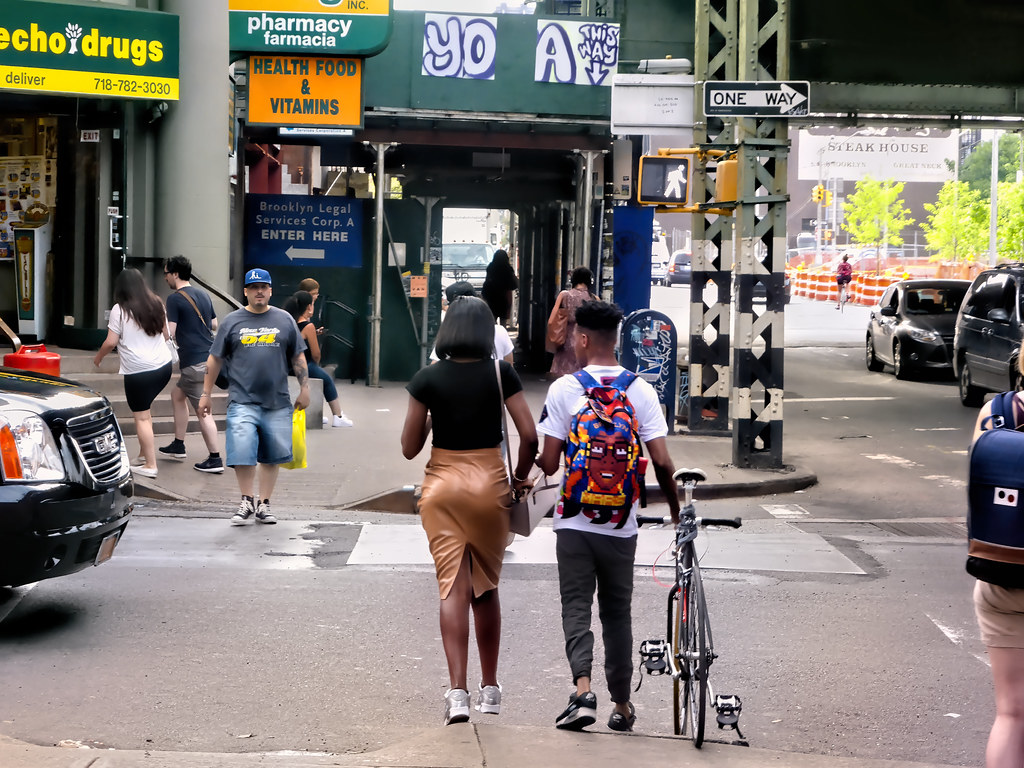In this nighttime photograph of a busy city street, the central focus is on a couple crossing the intersection hand in hand. The man on the right, dressed in a white t-shirt, gray slacks, and holding a bicycle in his right hand, wears a multicolored backpack with a pixelated design and a face, reading "Mars" below. Accompanying him on the left, the woman is seen in a black blouse, a gold skirt, white sneakers, and a light brown leather dress. To their left, another individual with a blue t-shirt and black sneakers is walking towards the camera. On the right side of the photo, another figure crosses with a backpack. The scene is bustling with activity, including several cars in the upper right, headed towards the camera, one being a black car and another an SUV, with trees visible above them. In the background, signs and storefronts line the street, including one indicating "Pharmacy or Pharmacia, Health Food and Vitamins" with a blue sign below, and another labeled "Echo Drugs, Deliver” accompanied by a phone number. Above the couple, a one-way sign and a walk signal are mounted on a pole at the intersection. The left edge of the image captures the front of another car, partially entering the frame.